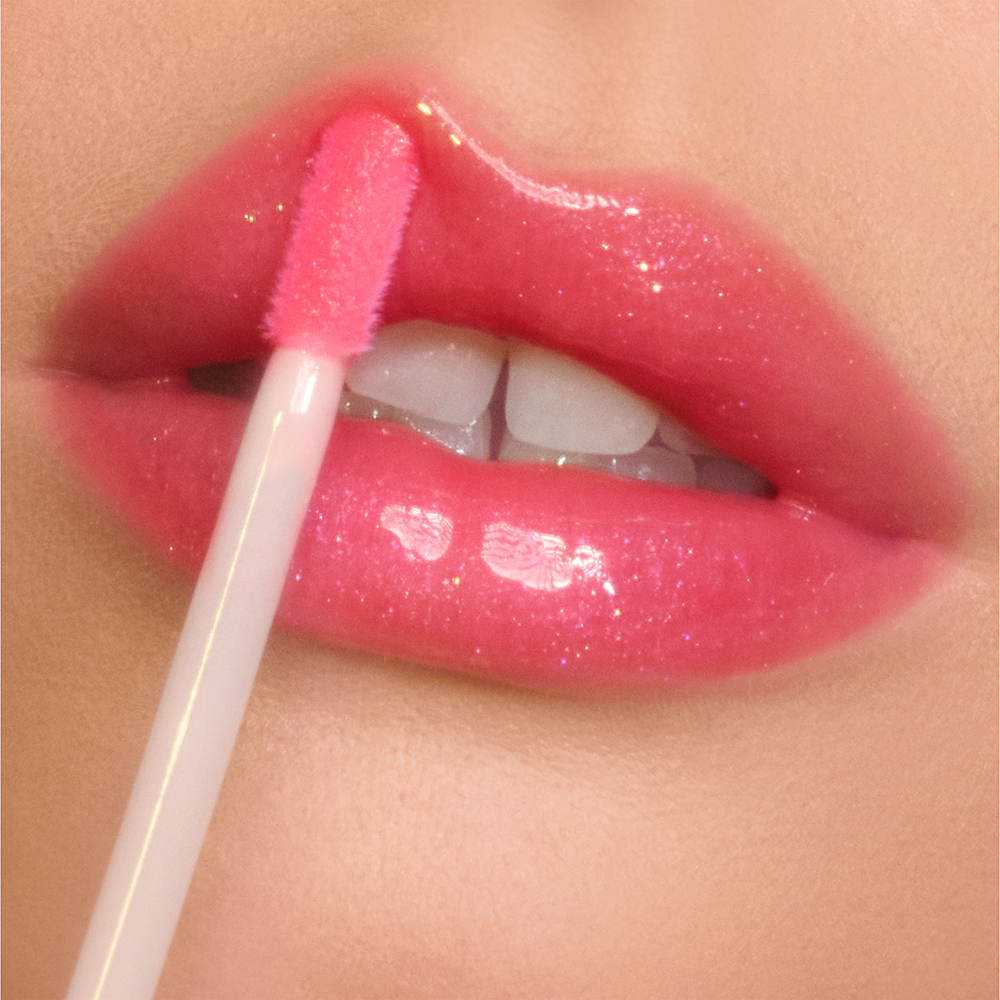This close-up photograph captures a fair-skinned individual, likely a woman, in the process of applying a vibrant, sparkly pink lip gloss to her lips. The glossy lips, highlighted by specks of sparkle, give off a radiant shine, particularly noticeable on the middle of the bottom lip. The gloss applicator has a white handle and a pink brush, matching the color of the lips but slightly lighter. The applicator is pushing up the left side of the top lip, causing a subtle distortion as it adds another layer of gloss. Beneath the lips, a few glossy, white teeth are partially visible through a slight gap. The focus remains tightly on the lips, with minimal visibility of the surrounding facial features, such as a hint of the chin and the area above the top lip.